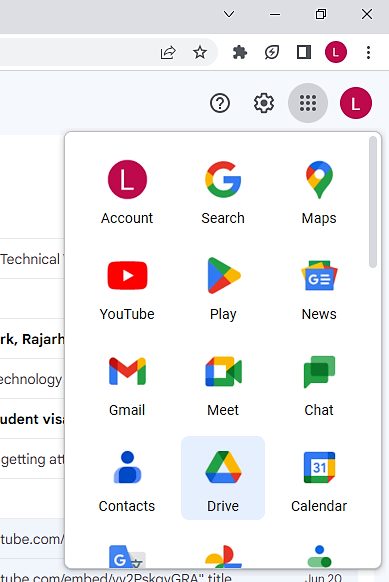The image depicts a user interface displaying a list of Google services and applications. The interface appears to be an app, likely accessed on either a mobile device or a computer. The layout suggests it is a web page or a settings menu within a Google account, featuring the user's initial prominently.

The visible services include:
- **Account:** The central hub for managing Google account settings.
- **YouTube:** The platform for video content.
- **Gmail:** The email service.
- **Contacts:** The address book for storing and organizing contacts.
- **Search:** The search engine functionality.
- **Google Play Store:** The digital distribution service.
- **Meet:** The video conferencing application.
- **Drive:** The cloud storage service.
- **Maps:** The navigation and mapping service.
- **News:** The news aggregator service.
- **Chat:** The messaging service.
- **Calendar:** The scheduling and time management application.

The interface is presented in a grid-like format, with each service represented by its respective icon, adorned with Google's signature colors. The user appears to be navigating through their Google account settings, possibly selecting a specific service from the menu to access further functionalities.